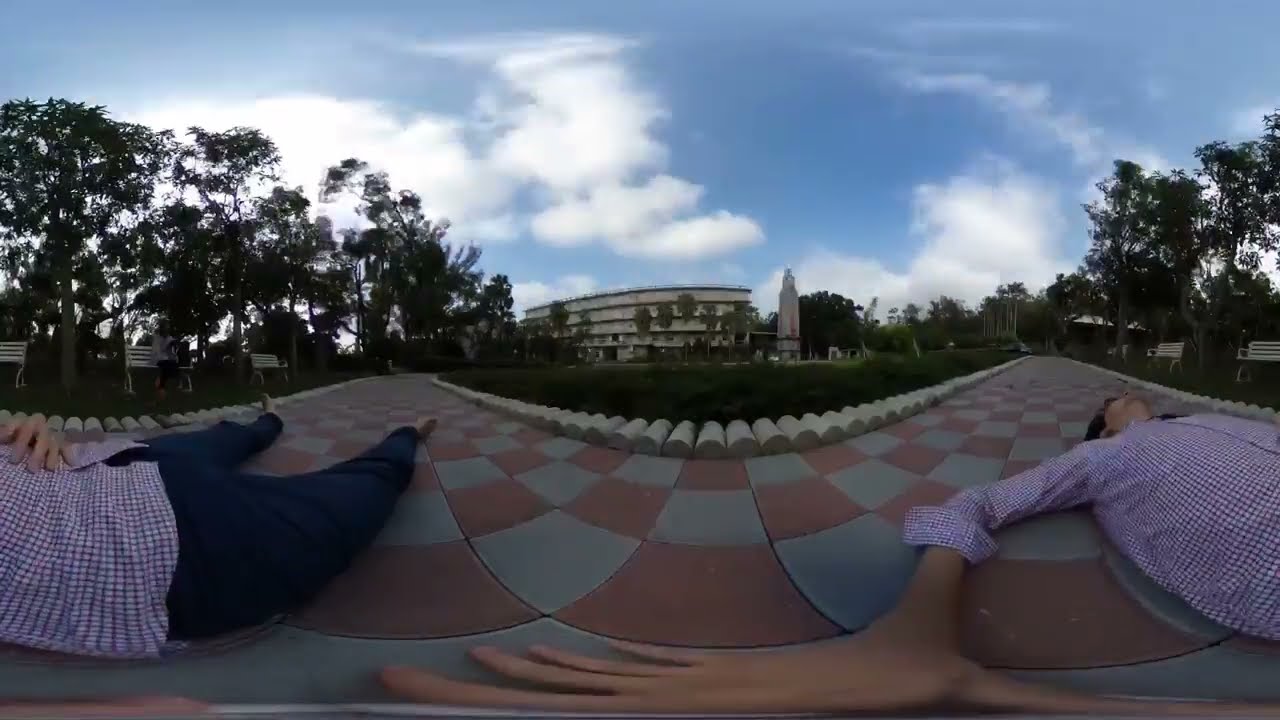The image captures a distorted outdoor scene on a cloudy day with patches of blue sky peeking through. The lens distortion creates an unusual visual effect, breaking a person's body into two parts. The lower half, legs and part of the torso, appear on the left while the upper torso and head are on the right, with the right hand stretched abnormally large at the bottom center, resembling exaggerated spaghetti-like fingers. The individual has black hair and wears a striped purple and black shirt. They lie on checkered flooring that features a mix of dark brown and light blue tiles, accented with small white bars. Surrounding this scene is vibrant green grass and trees on both left and right edges. An overexposed bit of cloud is visible in the upper left corner. In the background, a gray, rectangular, three- to four-story building and a small obelisk-like structure stand tall in the center, adding to the complexity of this peculiar and richly detailed outdoor image.